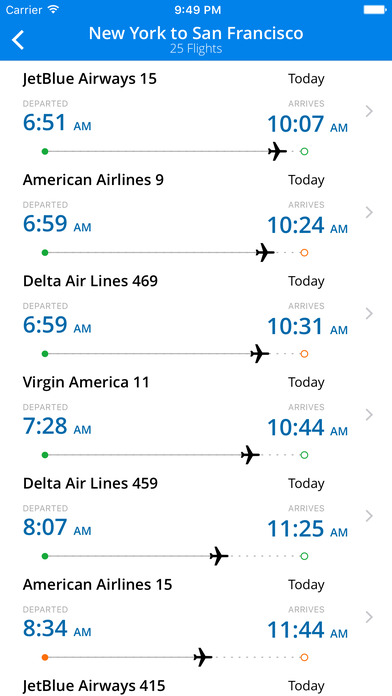This image depicts a flight schedule with a clean white background. At the top center, there is a blue header box that displays "Carrier" alongside the time "9:49 p.m." To the left of this header is a left arrow indicating a return option, and beside it, the route "New York to San Francisco" is specified, highlighting "25 flights."

Below this header, a list of flights to San Francisco from different airlines is presented, each accompanied by relevant details:
1. **JetBlue Airways 15** – Departed at 6:51 a.m., arriving at 10:07 a.m. This entry features a green dot connected by a line to an airplane icon, followed by another green dot.
2. **American Airlines 9** – Departed at 6:59 a.m., arriving at 10:24 a.m. Similar to the first entry, but ends with a red dot after the airplane icon.
3. **Delta Airlines 469** – Departed at 6:59 a.m., arriving at 10:31 a.m. It mirrors the format of American Airlines 9 with a red dot concluding the entry.
4. **Virgin America 11** – Departed at 7:28 a.m., arriving at 10:44 a.m. Features green dots at both ends with an airplane icon in between.
5. **Delta Airlines 459** – Departed at 8:07 a.m., arriving at 11:25 a.m. Similar to Virgin America 11, marked with green dots on both ends.
6. **American Airlines 15** – Departed at 8:34 a.m., with a unique sequence of a pink dot, dotted line, and red dot, concluding with a red end dot.
7. **JetBlue Airways 415** – Information on this flight is less detailed but follows similar symbol patterns as above.

Each flight entry concludes with a right arrow, indicating forwarding or next steps.